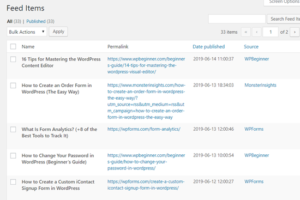The image depicts a user interface layout titled "Feed Items" in bold. It features selectable options with checkboxes next to each item, allowing users to either select all entries or only those marked as "Published." There is a pull-down menu labeled "Bulk Actions" with an accompanying "Apply" button for batch operations. 

The main section of the screen resembles a table format, displaying various items. Each row in the table starts with a checkbox on the left side, followed by the name of the item, which is presented with a blue hyperlink. Subsequent columns provide additional information, such as the date each item was published and its source.

Despite the image's small size and blurriness, it's clear that users can interact with the entries in multiple ways, including checking items individually or in bulk, searching through the feed via the search bar, and navigating through different pages of results to find specific content.